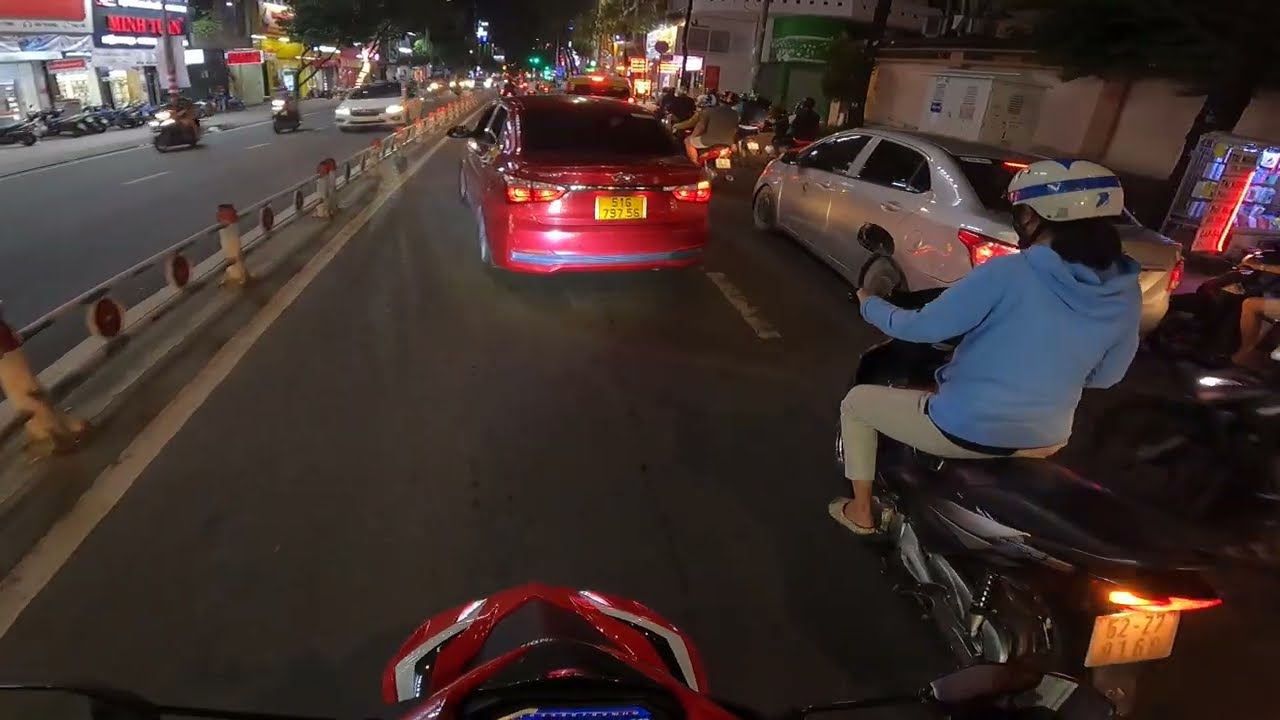The photo captures a busy urban street at nighttime from the perspective of someone riding a red and white moped. Directly to their right is another person on a black and silver moped, wearing tan pants, tan shoes, a blue hoodie, and a white helmet with a blue stripe. In front of the rider is a red car with the license plate 516-797-56, and to the right of the red car is a silver car. The street is congested with multiple mopeds and vehicles halted in a traffic jam. On the left side of the image, businesses line the streets with several mopeds parked in front of each establishment. Storefronts glow with lights and signage, illuminating the dark urban scene. A divider runs along the middle of the road, separating the lanes of traffic, which includes both motorcycles and cars. The sky overhead is dark, contrasting with the vibrant street activity below.